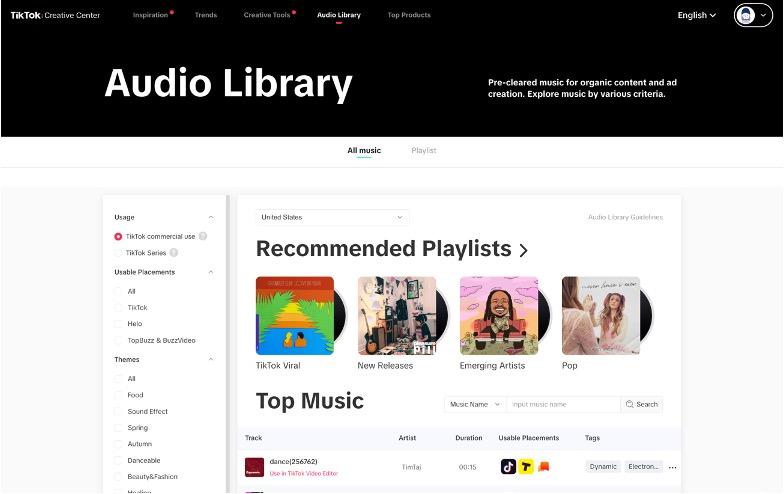**Description:** A detailed screenshot of the TikTok Creative Center's audio library interface. At the very top, within a black rectangular banner that spans the entire width of the screen, the words "TikTok Creative Center" are displayed prominently. Below this header, a navigation bar with the following options is visible: "Inspiration," "Trends," "Creative Tools," "Audio Library," and "Top Products." Also within this black banner, there is a subtitle that reads, "Precleared Music for Organic Content and Ad Creation, Explore Music by Various Criteria."

Beneath this banner, the layout divides into two primary white rectangular sections. On the left, a taller, vertically-oriented white rectangle appears. To the right of this, a shorter, horizontally-oriented white rectangle extends across the screen. The right rectangle is labeled "Recommended Playlist" and displays four album covers arranged side by side beneath this title. The album covers are categorized as follows: "TikTok Viral," "New Releases," "Emerging Artists," and "Pop."